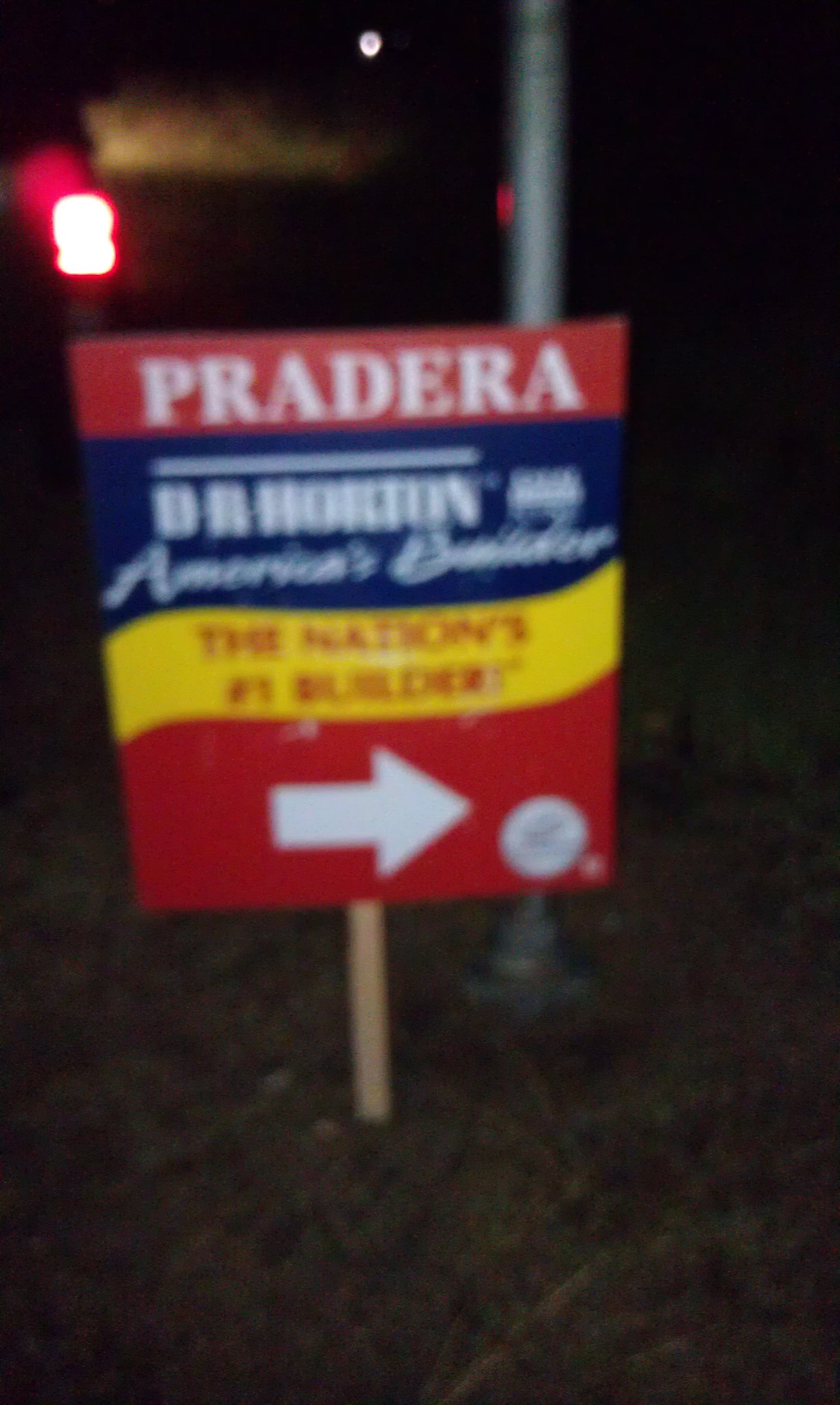This image depicts a blurry photograph of a large outdoor sign, likely taken at nighttime, planted beside a road and positioned in a grassy field. The sign itself is supported by a light brown wooden post and features several colorful sections with text. At the top of the sign, set against a red background, is the word "Pradera" in bold white letters. Below this, a blue section holds the text "D.R. Horton, America's Builder" in a combination of plain and cursive font. Further down, the sign highlights in red text against a yellow background, "The Nation's Number One Builder." The bottom section of the sign, which is red, displays a white arrow pointing to the right. Accompanying the sign is a metal pole nearby and a faint red light towards the back and left side of the image, adding to its overall out-of-focus and dimly lit quality.